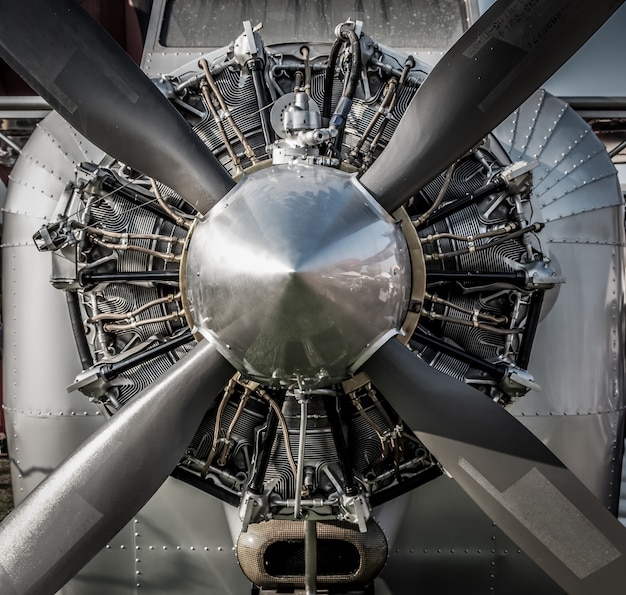The image is a close-up color photograph showcasing the front propeller of an aircraft. The aircraft's body is silver, detailed with silver screws holding the parts together and a see-through windshield showing some signs of precipitation. The reflective, chrome silver nose of the propeller houses four black blades. Surrounding the propeller are various metal components, including silver and bronze tubes connecting in different areas, and neatly arranged silver heat sinks behind the propeller fan resembling a network of heat exchanges. The smooth, meticulously designed machine displays an intricate assembly of metalwork, emphasizing the sleek, polished appearance of this part of the aircraft.